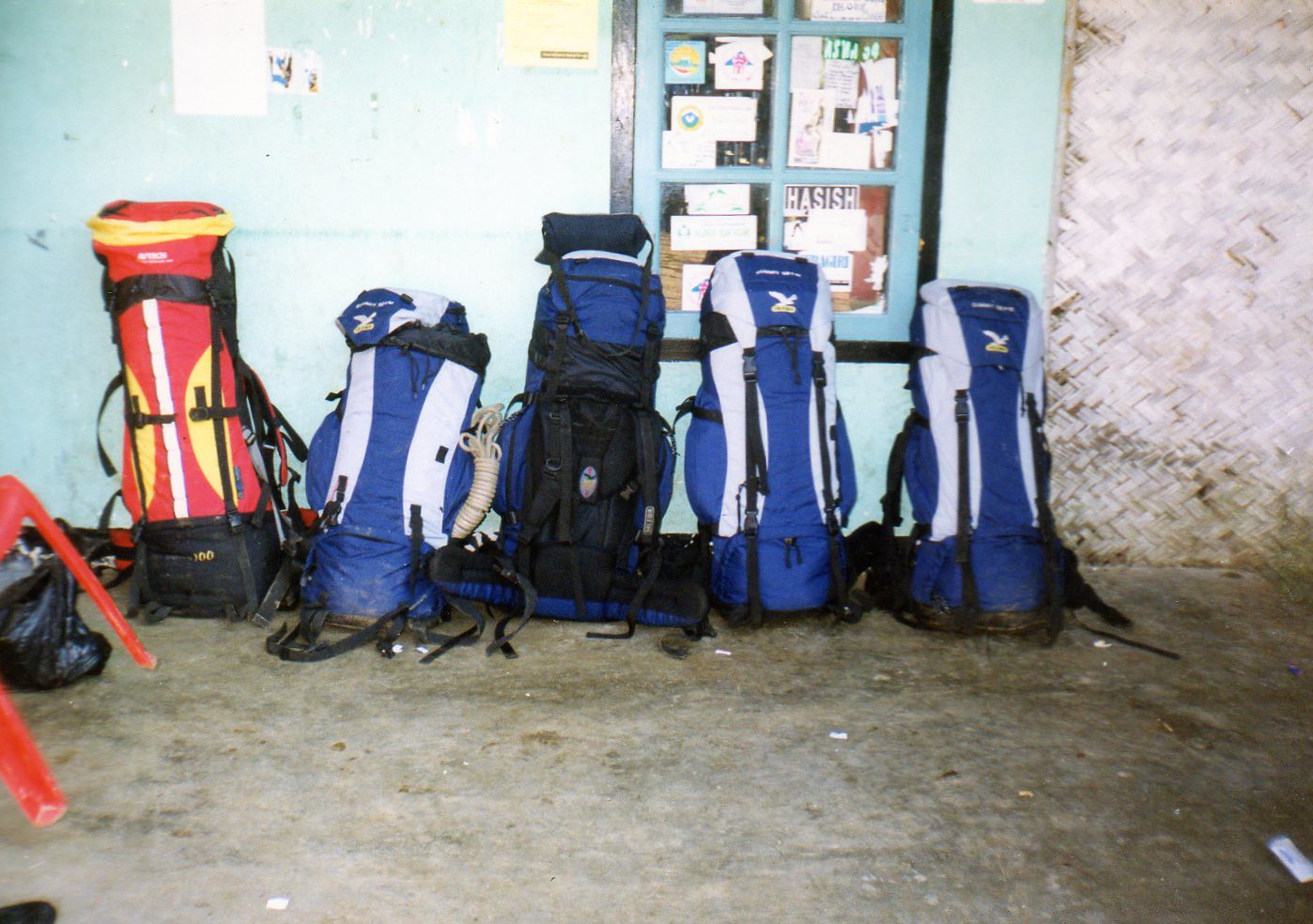This photograph captures an urban scene at night, highlighted by a flash, revealing a grimy, dirty concrete sidewalk where five large, tall backpacks are leaning against an exterior wall. The wall features two distinct textures: a section on the right is covered in tiles, while the rest is painted in an aqua teal plaster. A window, decorated in a darker teal blue with thick black trim, displays posters and stickers. Below, on the littered ground are various objects including a plastic chair and some scattered bags. Among the five backpacks, one on the left stands out in red with a black bottom and yellow trim. The remaining four are blue with white accents near the straps; three appear identical, and the fourth, also blue, has a rope tied to its side. Above the backpacks, a bulletin board covered in various advertisements adds to the cluttered ambiance. The overall scene is muted and desaturated, suggesting it wasn't taken on a sunny day but artificially illuminated for the shot.